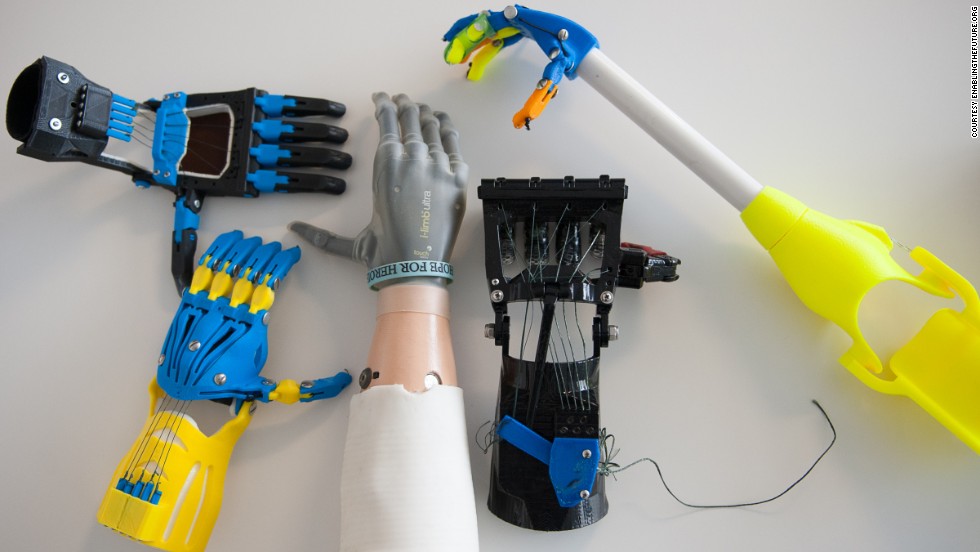This is a detailed color photograph depicting an assortment of five distinct robotic or prosthetic hands, arranged on a light gray, possibly whitish surface. Commencing from the upper left, the first object is a black robotic glove with blue joints at the knuckles, exuding a sleek and advanced technological appearance. Directly beneath it is another prosthetic hand, characterized by a longer yellow wrist section and blue fingers and palm, accentuated through yellow joints.

Transitioning to the middle of the image is a prosthetic arm designed for a more natural appearance, featuring a flesh-colored wrist transitioning to a gray plastic glove with a light blue band around it. Adjacent to this, towards the right, is a compact black prosthetic hand, with visible wiring and a blue section, possibly indicating an area for electronic connectivity.

At the extreme right, a device resembling a grabber or simplistic claw extends from the lower right edge to the center top of the image. This intriguing component has a blue, orange, and yellow hand-like ending attached to a long white tubular shaft, concluding with a yellow section that could correspond to an elbow joint. The entirety of these prosthetics showcases a predominant use of plastic materials, punctuated by metal screws, and features that could be 3D printed.